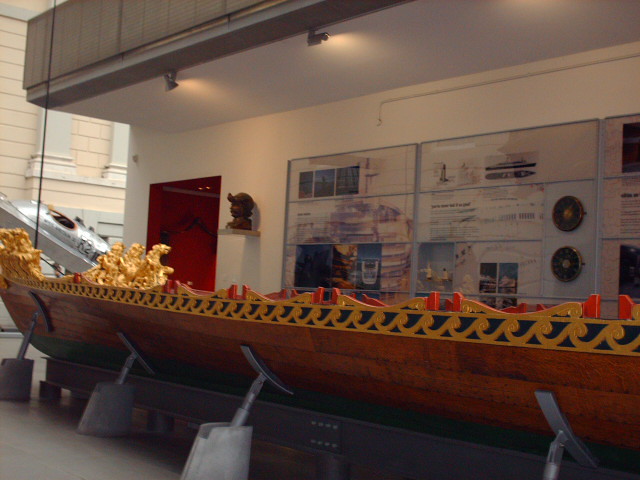The image depicts an interior scene, likely within a museum exhibit, featuring the façade of a long wooden boat prominently displayed at the center. The boat, which has intricate gold wave designs at its top, is supported by gray metal brackets. The background includes a white wall with a large information board behind glass, illuminated by two overhead spotlights. The floor is made of what appears to be hard linoleum. On the left side of the display, a doorway with a red interior and a bust hanging beside it can be seen. There's a large silver object and some signs in the left background, adding to the eclectic assortment of colors in the scene, which includes gray, silver, brown, yellow, orange, red, blue, and black. There are no people present in this neatly arranged exhibit, emphasizing the carefully curated and static nature of the museum setting.